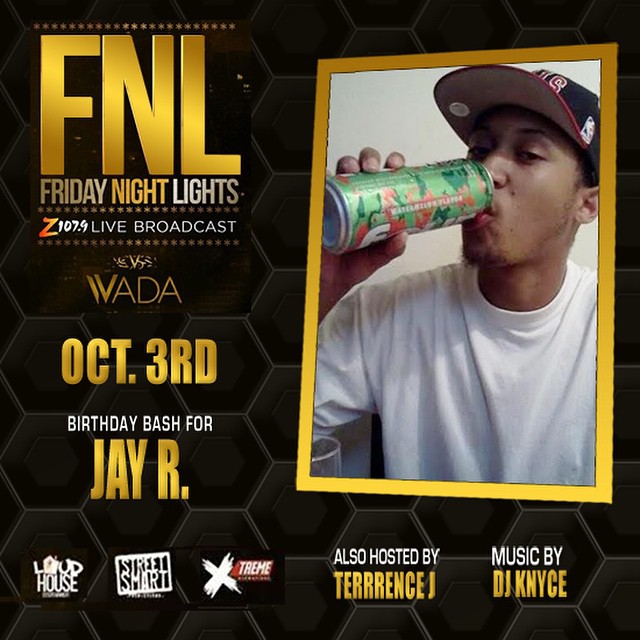The image is a promotional flyer designed with a black background featuring a honeycomb pattern in shades of gray for added depth. Dominating the upper left corner are large, golden text reading "FNL", followed by smaller text underneath stating "Friday Night Lights", "Z107.9 Live Broadcast", "VEDA", and then the date "October 3rd". Below this is a bold white text announcing "Birthday Bash 4", with the name "JR" highlighted in yellow text beneath it. 

The right side of the flyer is largely occupied by a photograph of a young, likely Hispanic man, happily drinking from an energy drink can. He is wearing a white shirt and a blue and red cap, holding the can up to his lips with his right hand while facing the camera. 

At the bottom right, in white text, it says "Also Hosted By", followed by the name "Terrence J" in yellow text. Adjacent to this, in white text, it mentions "Music By" with the DJ's name "DJ KNYCE" in yellow text. Additionally, the bottom section features five logos, with three on the left and two on the right corresponding to the host mentions.